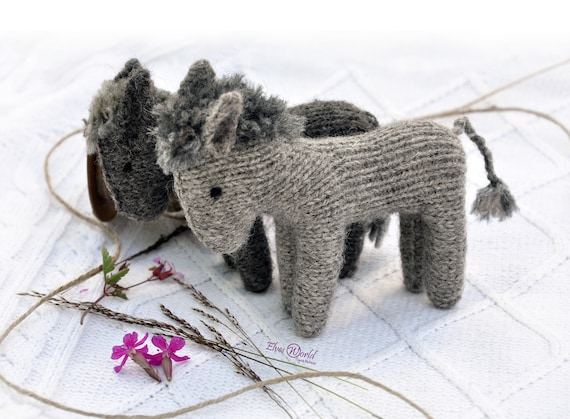The photograph features two hand-stitched, crocheted donkeys standing on a blue and white checked fabric surface. The donkey in the front is a light gray with a darker gray mane and tufted tail, its ears perked and its mouth pointing down. Behind it, a slightly smaller, darker gray donkey with a similarly tufted tail and bushy head of hair is visible. Both donkeys have black eyes and adorable features. Scattered around them are a few dried flowers, some purple in color, and a piece of jute twine draped across the fabric. A small watermark that reads "Elva's World" indicates the creator of these charming stuffed animals.